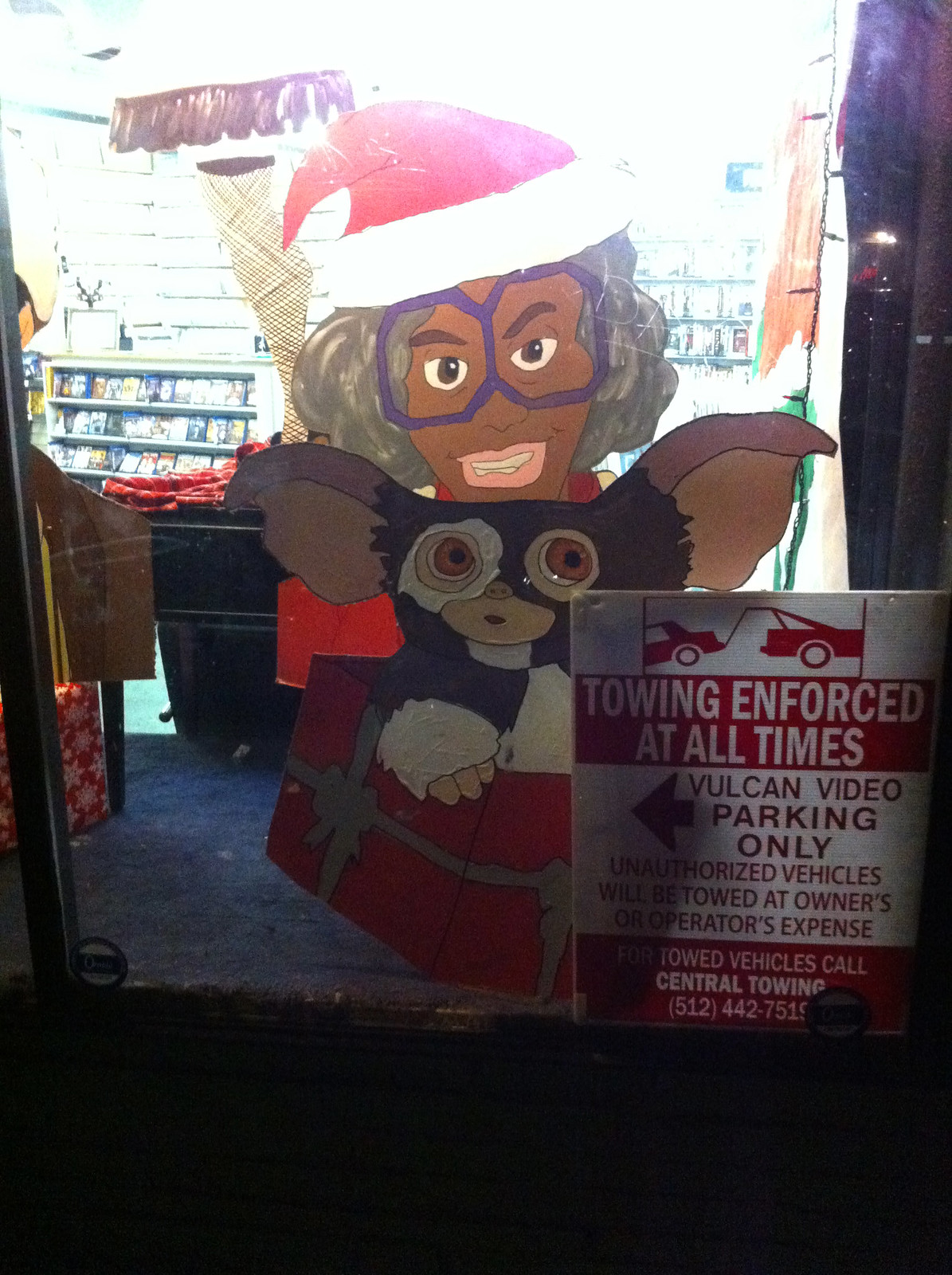The image is a color photograph taken outdoors at night, capturing the storefront window of a shop. The view is from the perspective of someone standing on the street, looking inside. Prominently displayed on the window is a detailed sign that reads, "Towing enforced at all times. Vogue in Video parking only. Unauthorized vehicles will be towed at the owner's or operator's expense. Towed vehicles call Central Towing 512-442-7519," with an illustration of a vehicle being towed. Above the sign, there's a vibrant painted image featuring two figures: a black woman with brown skin and bold purple eyeglasses, smiling warmly at the viewer while wearing a Santa Claus hat, and below her, a gremlin-like creature with large ears, emerging from a red gift box. The interior of the store is bathed in low light, revealing shelves filled with DVDs. The walls are lined with Christmas decorations, including streamers hanging from the ceiling and lights, adding a festive atmosphere to the scene. Although it is dark outside, the store is well-lit, providing a cozy, inviting glimpse into the shop's interior.